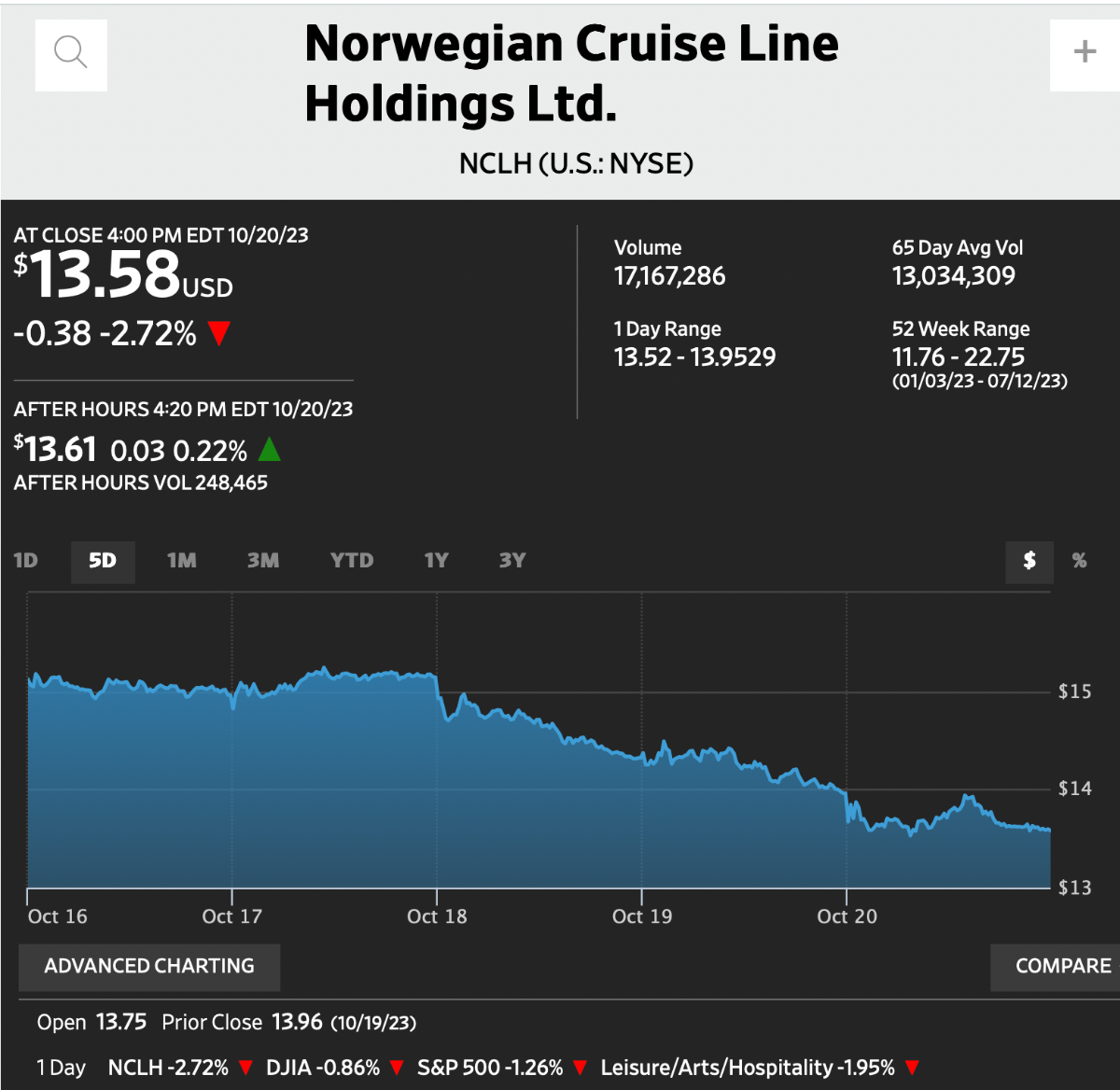This image depicts a detailed view of the Norwegian Cruise Line Holdings Ltd stock performance on the New York Stock Exchange (NYSE). Prominently displayed is the company's name in black letters, with its ticker symbol 'NCLH' in parentheses, indicating its listing on the US exchange in New York City. A white square with a magnifying glass icon, presumably for searching, and a plus sign are visible on the left corner of the image.

As of the market close, the stock price is shown to be $13.58 USD. Additionally, after-hours trading indicates a slight increase to $13.61 USD, reflecting a 0.22% rise. A blue bar graph at the bottom charts the stock's performance over a five-day period from October 16th to October 20th, with the graph showing a decline from about $15 on October 16th to the $14 range by around October 20th.

The image includes several charting options for different time frames: one day, five days, one month, three months, year-to-date, one year, and three years, highlighting the advanced charting capabilities. On the right side of the graph, dollar markers for $15, $14, and $13 are displayed. The stock's previous close was marked at $13.96 and the opening price at $13.75. The background is all black with white lettering and numbers, while the bar graph is depicted in a baby blue color.